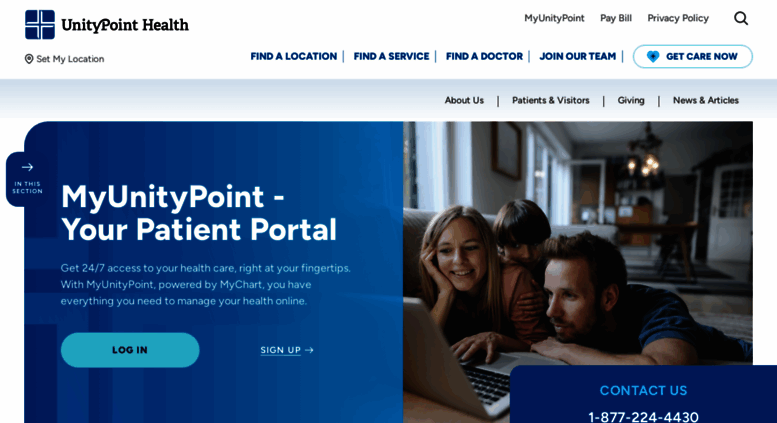This screenshot captures the homepage of the UnityPoint Health website. In the upper left-hand corner, the UnityPoint Health title is prominently displayed alongside their logo, which features a blue square with a white cross. To the right of the logo, the main navigation menu offers options such as "Find a Location," "Find a Service," "Find a Doctor," and "Join Our Team."

Dominating the main portion of the page is a heartwarming image of a family scene: a man, a woman, and a young boy crouching in front of a couch, engrossed in something on a laptop computer. To the left of this image, white text reads "MyUnityPoint, your patient portal." Below this text are two action buttons—for logging in and signing up—offering users quick access to the patient portal.